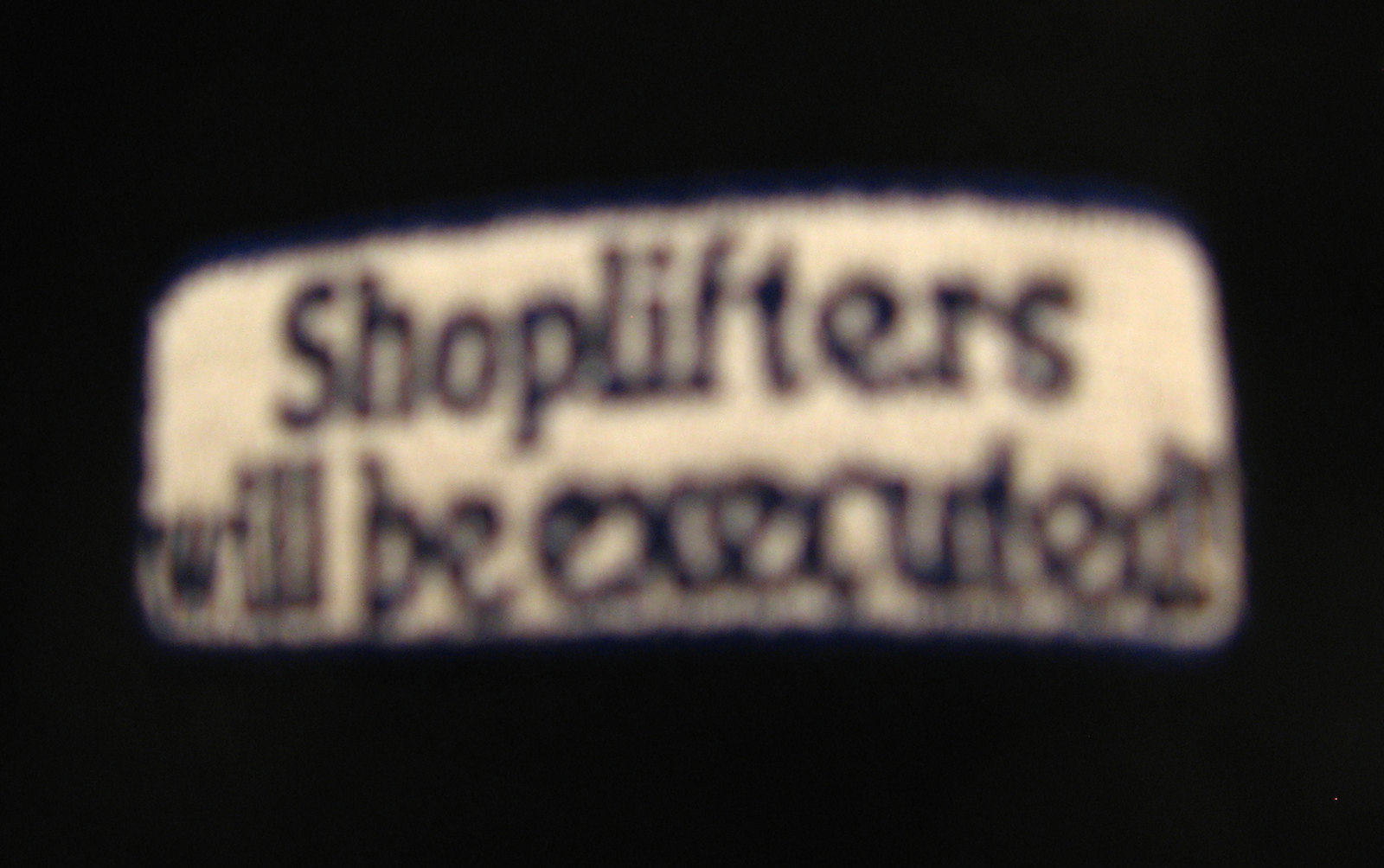This photograph appears to have been taken with a low-quality camera, resulting in a very blurry and grainy image. The background of the photo is completely black, which makes the central image stand out prominently despite its blurriness. The central image is a white rectangle, possibly a patch, sign, or marquee, with curved edges. The text on this white rectangle is rendered in what might be navy-colored, embroidered thread, though the blurriness makes it hard to distinguish the precise color and details.

The text itself is quite legible due to its size and contrast against the white background. It reads, "Shoplifters will be executed," with "shoplifters" on the top line and "will be executed" arranged beneath it in two rows. The only capital letter is the 'S' in "shoplifters." The border of the rectangle also appears to be in a navy or lighter navy color, but this is not entirely clear due to the image's poor quality. The black background and the simple yet striking message create a stark and somewhat ominous visual effect.